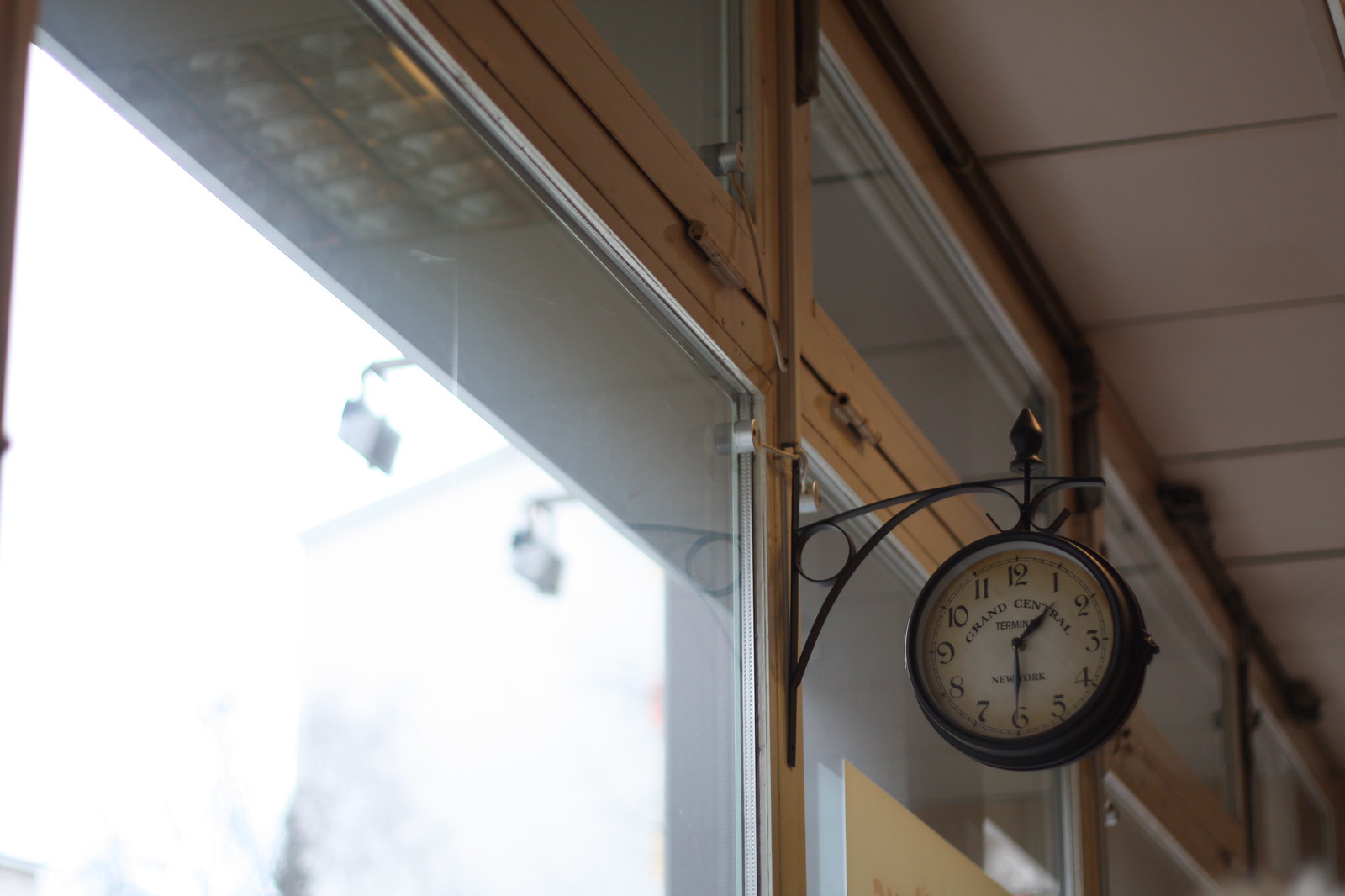In the image, we see a detailed view of the upper edge of a glass wall within a corridor, bathed in abundant daylight streaming through numerous windows. Prominently hanging on a vertical strut supporting the glass windows is an ornate vintage-style clock. The clock, set to 1:30 p.m., features a round face with classic black numbers, a black exterior, and a white interior with the inscription "Grand Central Terminal" and "New York" below it. The clock is mounted on an elaborate metal bracket adorned with intricate circles, angles, and a pointed top. The ceiling above consists of modular panels and sections, with visible utilities such as wires and cables where the glass wall meets the ceiling. Additionally, an outside awning area with lights shines back towards an unspecified sign, creating a well-lit and dynamic backdrop. The design of the windows and their frames includes an orange taupe hue, adding a touch of color to the scene. The overall ambiance hints at a setting reminiscent of a train station or a railway terminal.